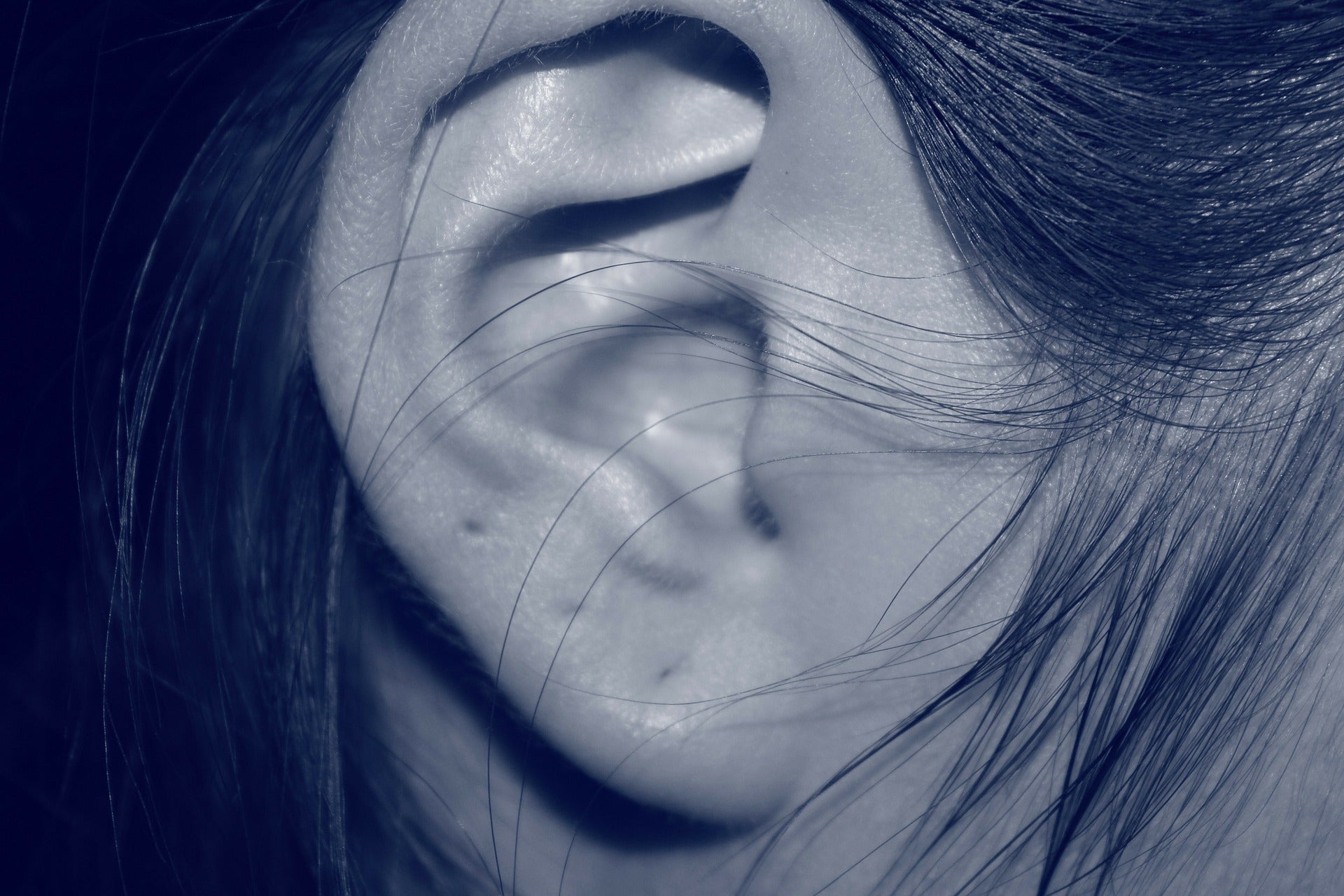This close-up photograph features a relatively small, feminine right ear, filtered with a blue overtone. The ear, devoid of any remarkable features, is surrounded by wisps of dark, likely black hair, which are both in front of and behind it. Notably, the hair is pulled behind the ear, with a few strands still draping over the top and in front. The ear lobe reveals evidence of three piercings, which appear to have mostly healed and closed up. The image is zoomed in enough to display the hair follicles along the outer shell of the ear and a shadow cast on the lobe at the bottom. A potential small freckle is visible within the hair follicles to the right of the ear. The inner part of the ear remains obscured, maintaining focus solely on the ear’s exterior.